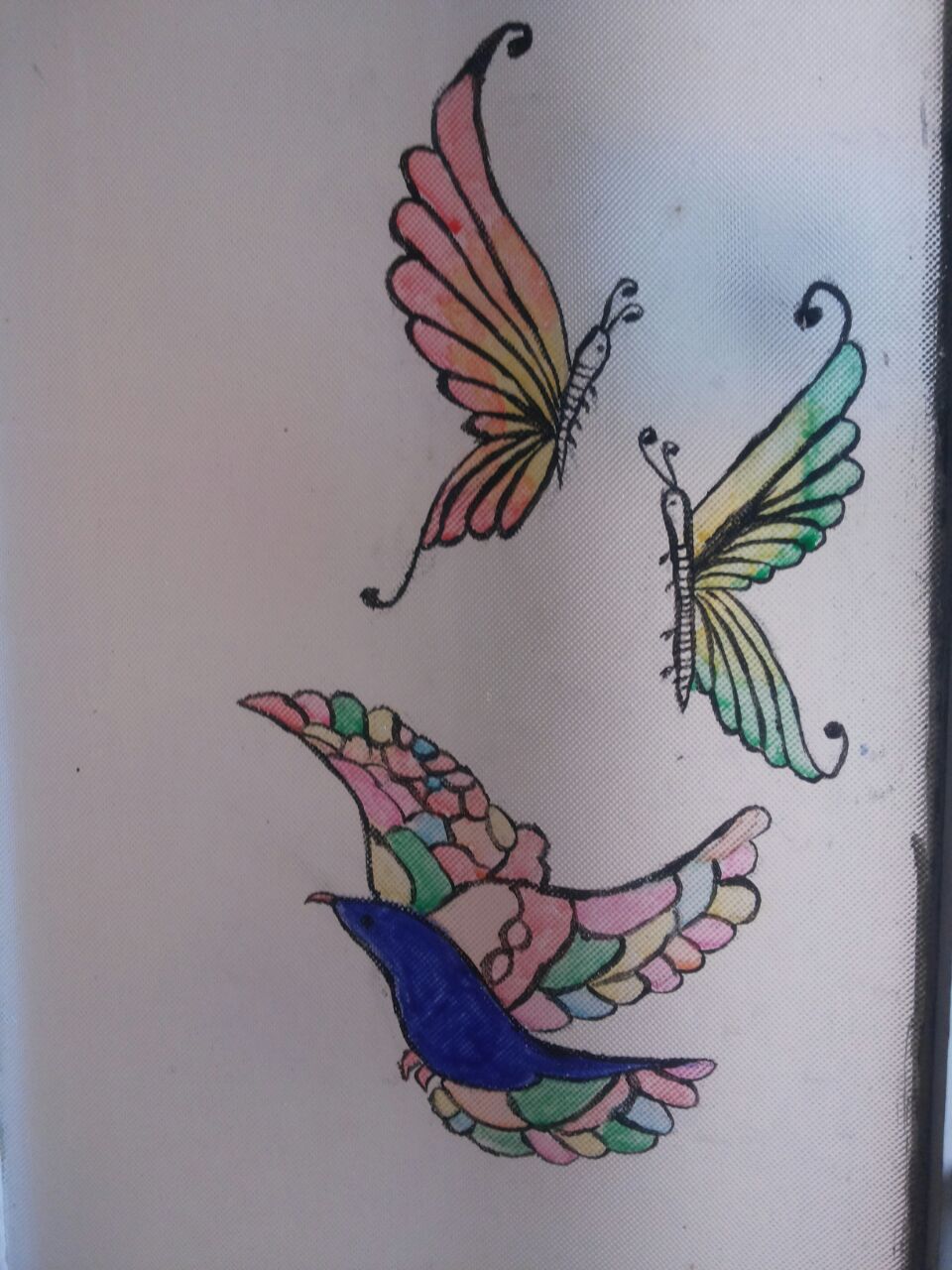The image features a light purple paper background adorned with three distinct butterflies, each showcasing its own unique beauty. 

The top butterfly boasts a slender, elongated body with two delicate antennae, and a slightly curved, tiny black tail. Its wings, a vibrant blend of orange and yellow, stand prominently, exuding a captivating allure.

The second butterfly has a long, thin black body adorned with two fine antennae. Its wings exhibit a gentle amalgamation of greens and yellows, creating a soothing and graceful appearance.

The third butterfly, a true spectacle of color, displays a myriad of hues: red, pink, green, yellow, blue, and brown. Intriguingly, at the center of this butterfly’s multicolored wings, rests a large, striking blue bird, adding an unexpected and enchanting element to the overall composition.